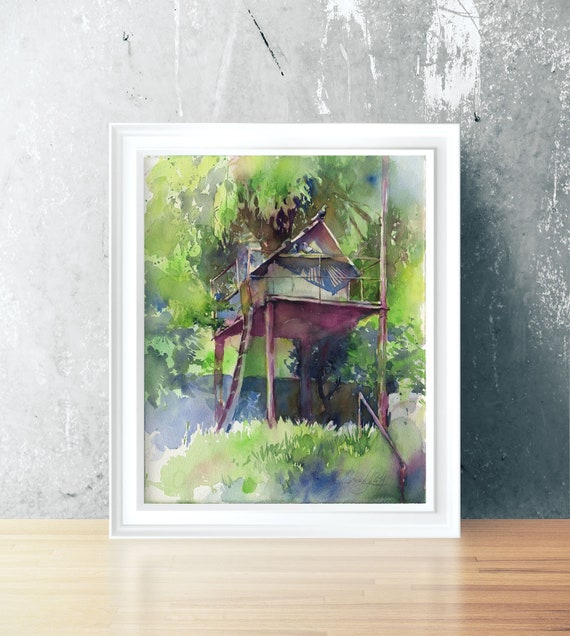The image showcases a detailed watercolor sketch of a treehouse, elegantly framed in a white border approximately an inch to an inch and a half wide. The artwork leans against a silver-gray wall that features white splatter marks, reminiscent of a painter's studio. The floor beneath is a light bamboo beige, providing a subtle contrast to the vibrant hues of the painting. 

The treehouse itself is elevated on large poles and accessed by a ladder. The structure has an A-frame roof with windows at the front, evoking a quaint, whimsical charm. Surrounding the treehouse, green and yellow leaves dominate the scene, with bleeding edges in various shades of green, yellow, and blue, giving it a fluid, dynamic feel. 

Additional details include sparse green leaves sprouting from a bush area at the bottom and the treehouse's elements tinted with purples and blues. The overall effect of the painting is one of ethereal beauty and serene outdoor escapism, captured in the delicate, flowing strokes characteristic of watercolor artistry.